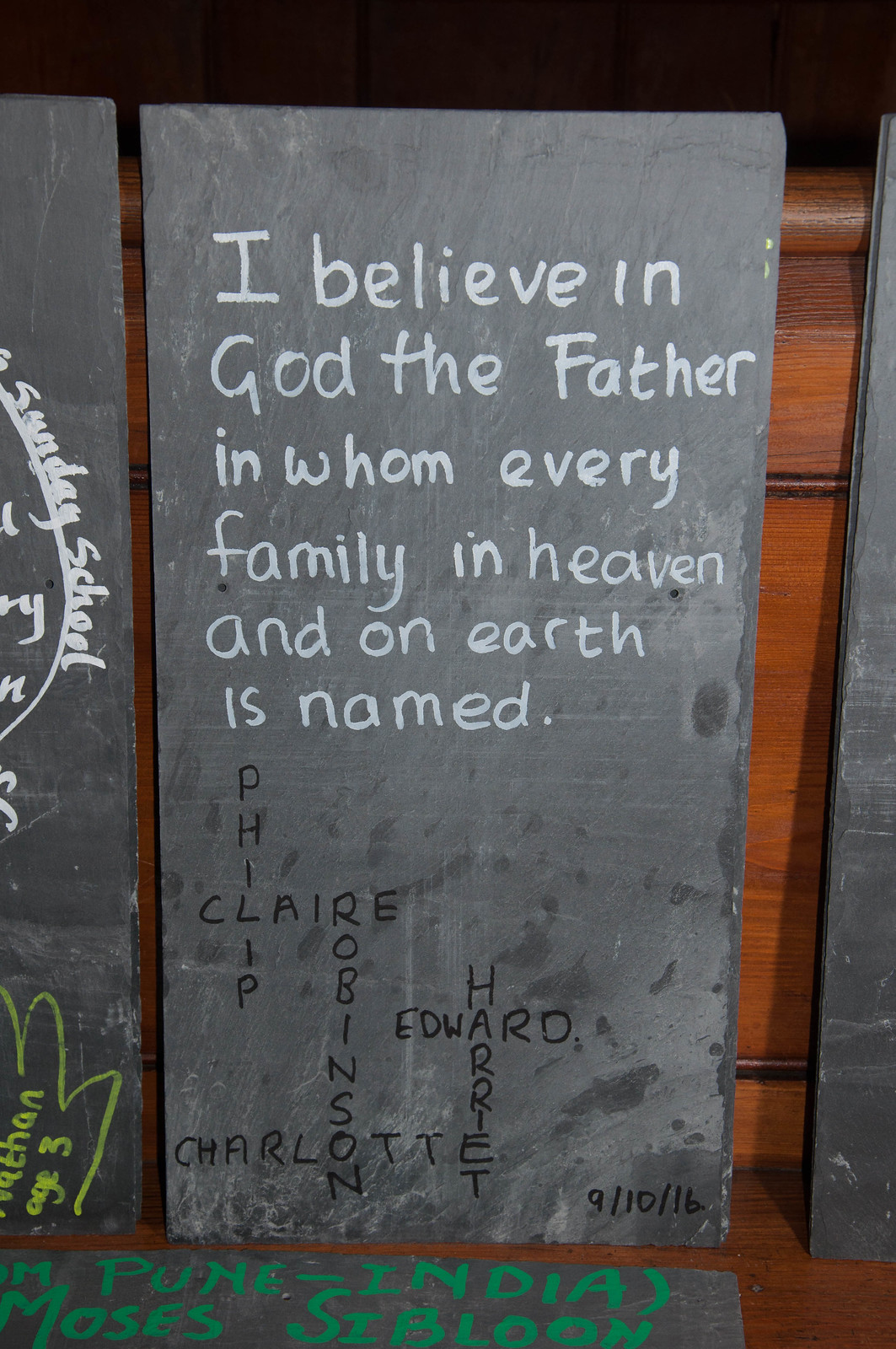This is a tall, rectangular image of a sign that appears to be like a chalkboard, set against a surface made of dark brown, fancy-looking wooden slabs. The sign, positioned between two similar ones, is resting on a wooden surface. It features a dark gray rectangular background with white chalk text at the top that reads: "I believe in God the Father in whom every family in heaven and on earth is named." 

Beneath this proclamation, several names overlap in black handwriting, creating a design reminiscent of a crossword puzzle. The names include Philip (written vertically), Clare (written horizontally intersecting the "L" in Philip), Robinson (starting with the "R" in Clare), along with additional names like Charlotte, Edward, and Harriet. The chalkboard shows some dirt marks and what appear to be wet splashes near the bottom, adding to its rustic look. The date September 9th, 2016, or September 10th, 2016, is noted, suggesting when it was written. The lower edge of the image features some text: "poon india moses cibloon" in green, although not fully clear. Additional chalkboards or plaques are visible on either side, but they are cut off at the bottom.